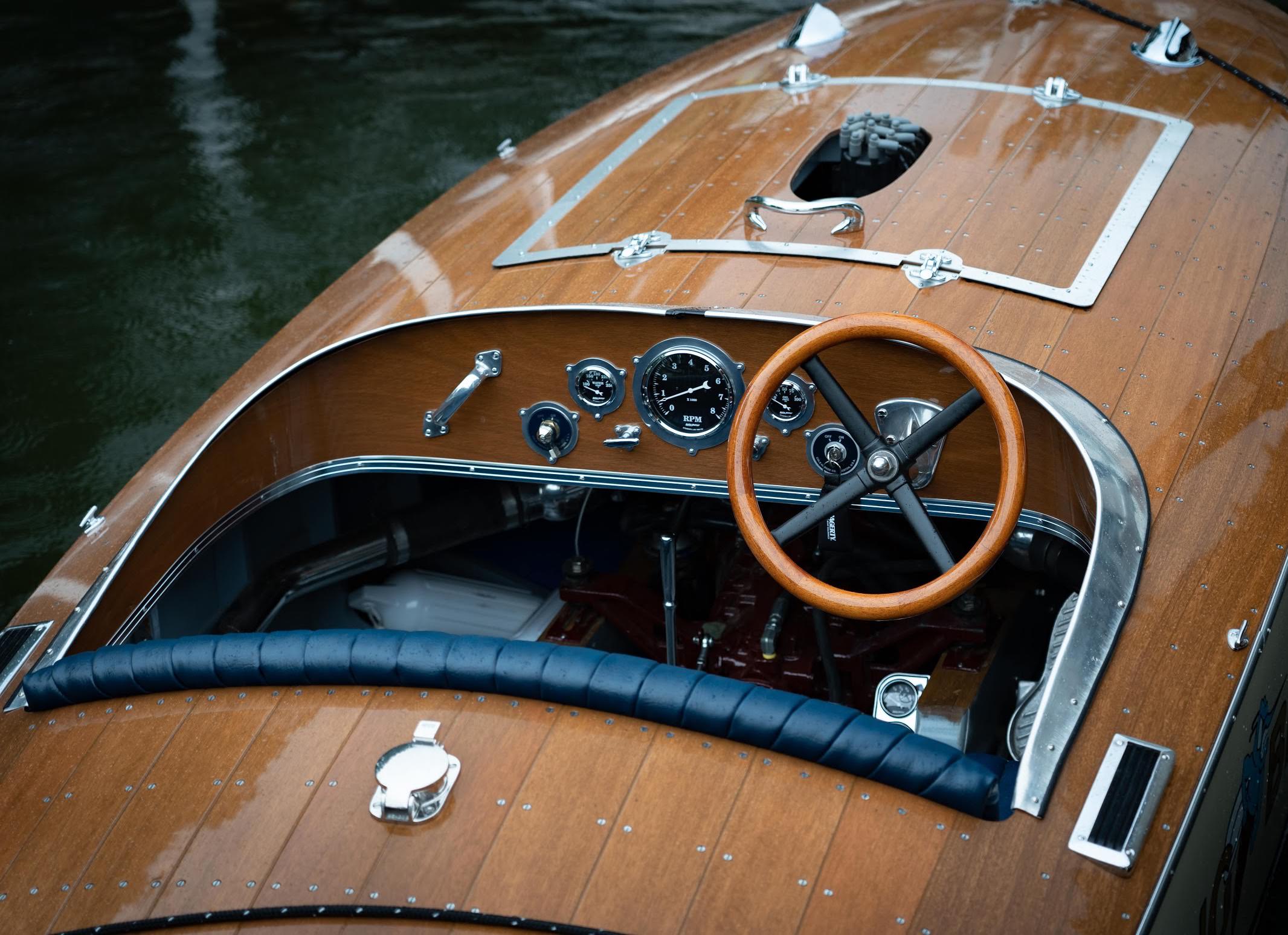An overhead view captures a vintage wooden speedboat on slightly murky green-gray water, reflecting some light yet appearing shallow. The visible front two-thirds of the boat showcases its glossy, possibly mahogany, panels. The boat exhibits a classic design with a meticulously maintained and polished appearance. The dashboard, lined with silver gauges on a black background, includes a variety of dials, one scaling from zero to eight, and several knobs and pedals. A brown steering wheel with black supports is prominent. The dashboard also features a gray metal handle and a possible gear shifter. In the seating area, two blue-vinyl bucket seats rest atop a predominantly wooden interior, with adjacent silver running lights. Behind the seats, a metallic access hatch or fuel cap is visible. The boat's elegant design is underscored by a visually striking cream-colored side, confirming its timeless beauty.